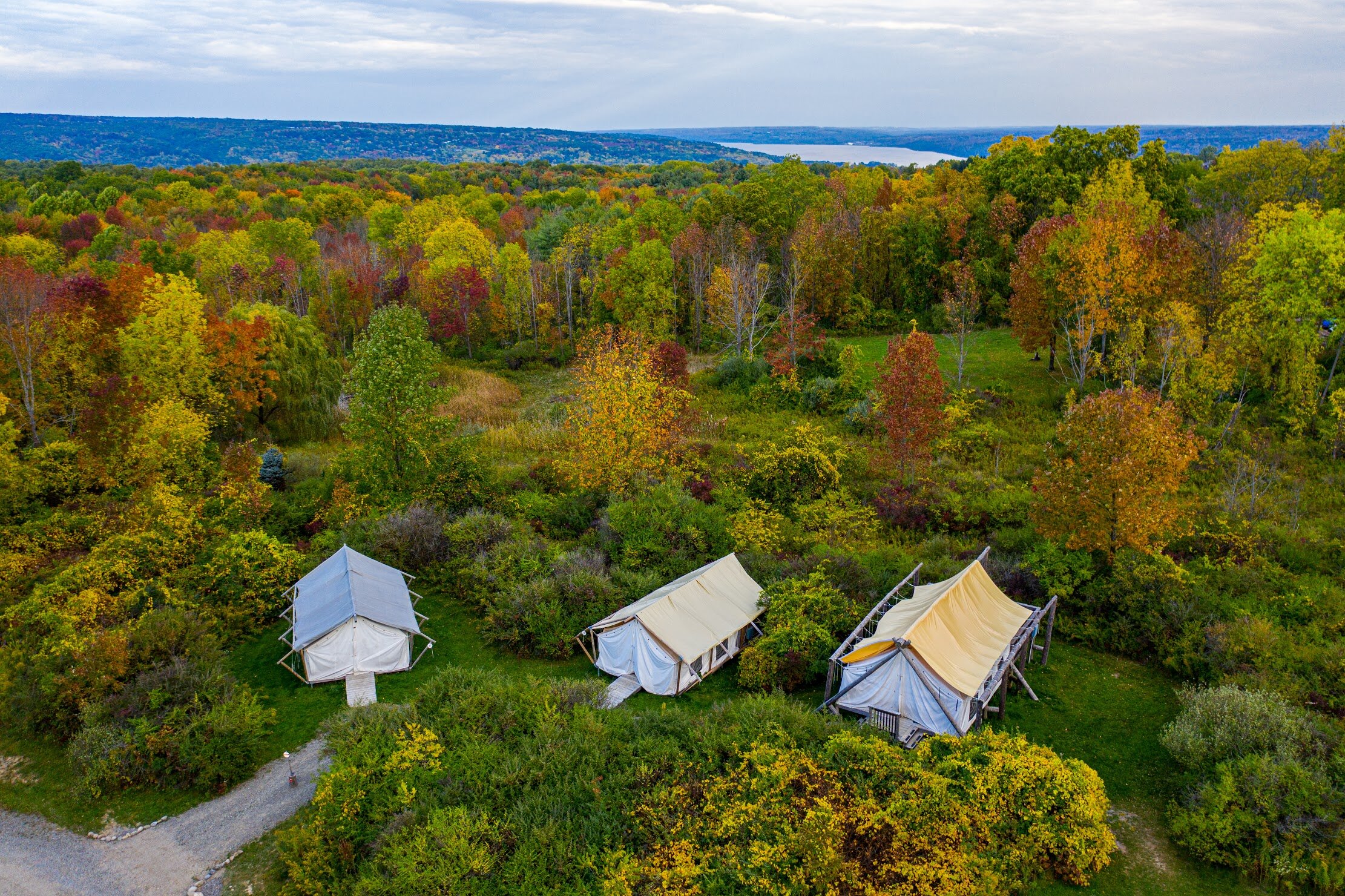The image captures a serene autumn campsite in the middle of a dense forest, viewed from a high vantage point. Three large, barn-shaped tents are prominently situated in the center, each distinct in color: the first tent on the left has a white body with a gray roof, the middle tent features a white body with a pale beige roof, and the largest tent on the right boasts a white body with a bright yellow roof. Surrounding the tents at the forefront is a mix of yellow and green brush, lending a lively contrast to the scene. Behind the tents, the forest displays a vibrant array of autumn foliage in various stages, with leaves glowing in hues of yellow, red, orange, and green. Beyond this colorful treeline lies a small river and even more trees fading into the distance, predominantly green due to their remoteness. The sky above is overcast but pierced by rays of sunlight, suggesting daytime under a cloud-filled canopy. A sense of tranquility permeates the lush, relaxing environment, highlighting the natural beauty of the season.